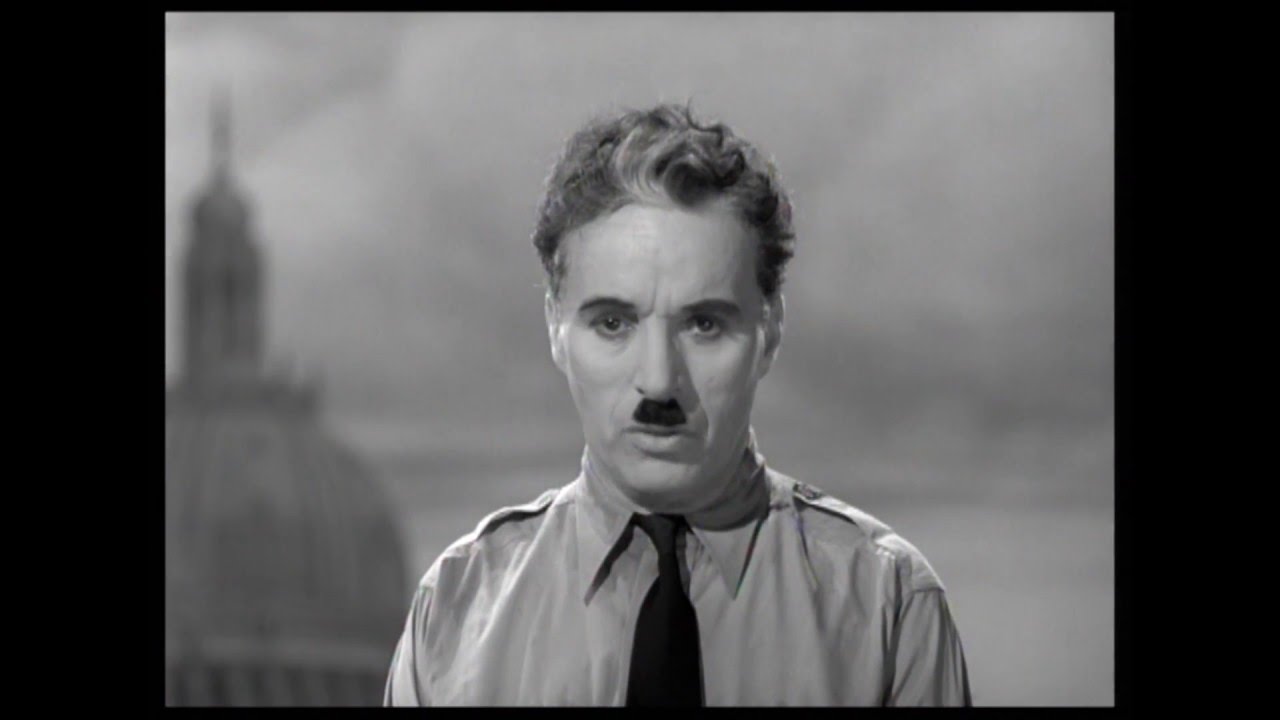The image is a black and white photograph featuring a man with a mustache reminiscent of Adolf Hitler or Charlie Chaplin, creating an evocative, almost cinematic effect. The photo is framed by thick black borders on the left and right, and thin black borders on the top and bottom. The man, who bears distinctive eyebrows and a fair complexion, has short-cropped curly hair with a noticeable white widow's peak. He is dressed in a collared, button-up shirt with lapels on the shoulders, suggesting a military style, and he wears a black tie.

The man's gaze is directed slightly off-camera, adding a sense of contemplation or melancholy to his expression. The background is blurry but shows a large, impressive building with a rounded roof, a turret, and a long or tall steeple area, set against a sky filled with grey clouds. This setting contributes to the historic and somewhat somber tone of the photograph. The overall aesthetics and elements suggest this could be a still from an old movie or a dramatic portrayal.